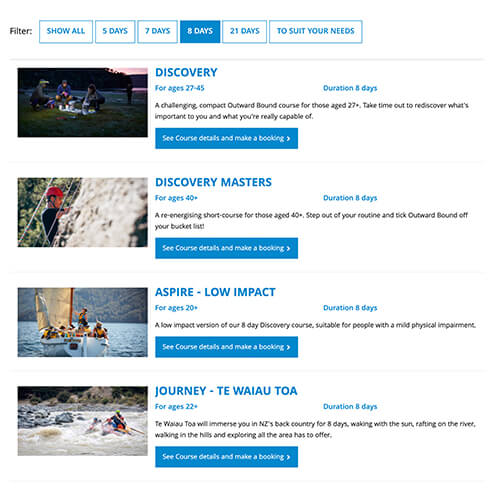The image is a screenshot of what appears to be a travel booking platform. At the top left corner, there's a section labeled "Filter." The filter options include durations such as "5 days," "7 days," "8 days," and "21 days," allowing users to choose the length of their trip to suit their needs.

The main part of the screenshot is divided into different sections, each presumably offering a unique type of travel experience:

1. **Discovery**: This section features an image of a scenic beach at nighttime.
2. **Discovery Masters**
3. **Aspire**
4. **Low Impact**
5. **Journey to Waiwotoa**: This section includes an "Ages" category, indicating that the trips may have age-specific recommendations or restrictions.

Each section seems designed to cater to different interests and preferences, allowing users to explore a variety of travel experiences.